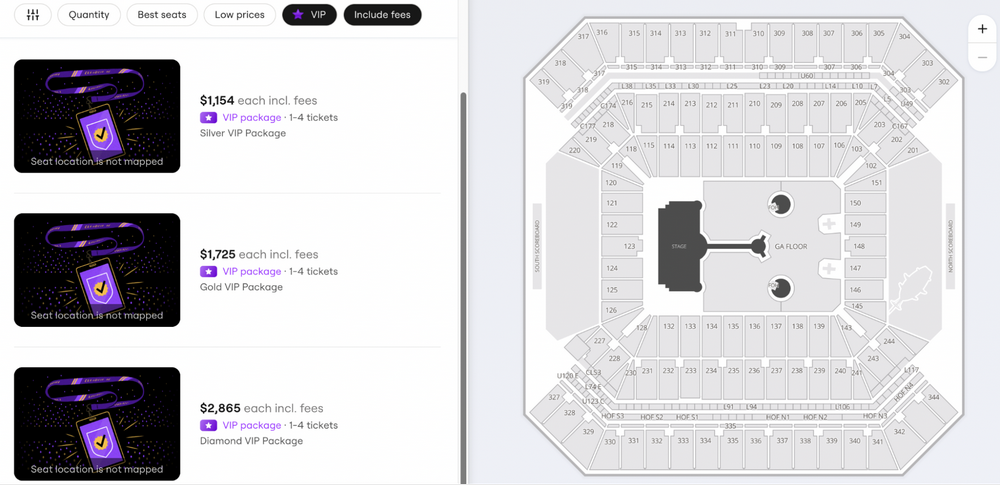This detailed image is a seating chart for an event, visually depicting the stage location and the arrangement of seats divided into sections numbered in the 100s, 200s, and 300s. The diagram is color-coded and clearly marks various seating options and their corresponding numbers.

On the right side of the image, there is an informational sidebar that highlights important purchasing options. This sidebar includes filters for "Quantity," "Best Seats," and "Low Prices," all shown in white buttons, as well as "VIP" and "Include Fees," both shown in black buttons. This section also specifies different VIP packages available for purchase. 

The pricing details are as follows:
- Silver VIP Package: $1,154 each, including fees, with options for 1 to 4 tickets.
- Gold VIP Package: $1,725 each.
- Diamond VIP Package: $2,864 each.

Notably, the seat locations for these VIP packages are not mapped on the chart. Additionally, the image displays a purple VIP pass with black boxes, which is presumably something you can wear on a lanyard around your neck.